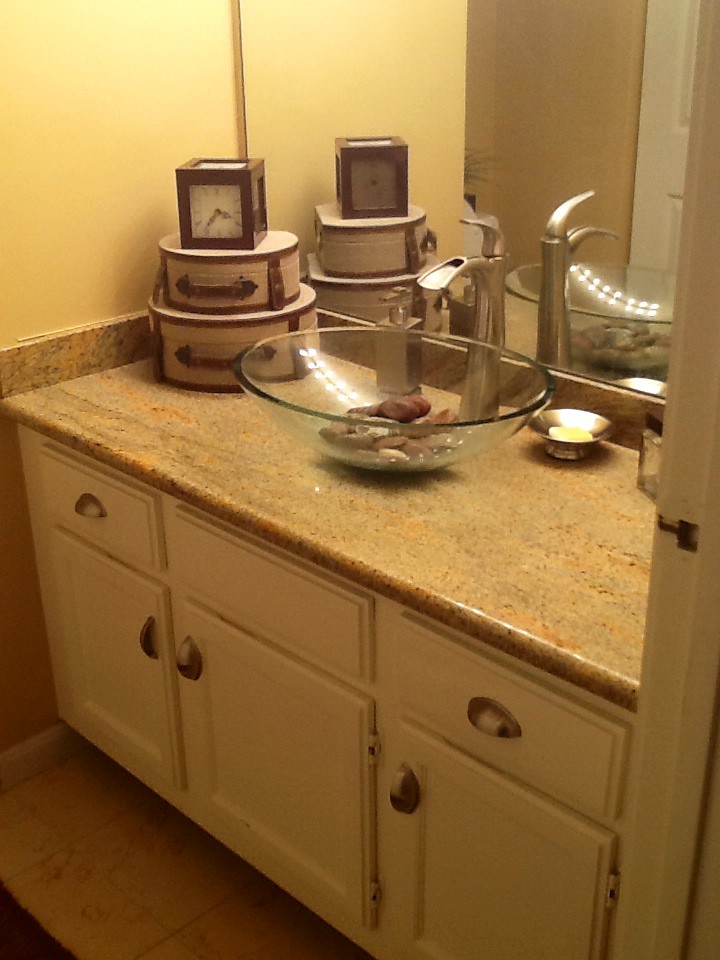The photograph captures an elegant bathroom sink area with yellow walls creating a warm ambiance. A large mirror spans the back of the sink area, reflecting the room's stylish elements. The countertop, designed to mimic marble, showcases a rich brown color accented with orange and deeper brown striations. Atop the counter sits a distinctive glass sink bowl, elevated rather than sunken in. The bowl intriguingly contains rocks, adding a rustic touch.

In one corner of the countertop, two cream-colored hat box-style storage boxes with brown detailing and handles are neatly stacked. A small, cube-shaped clock rests on top of these boxes, adding a touch of modernity. Centrally placed behind the sink is a faucet with an antiquated, hand pump design, evoking a charming, old-world feel. To the side, a silver dispenser, likely for soap, stands next to a matching silver soap dish holding a piece of yellow soap.

Below, the cabinetry comprises white drawers and doors, each adorned with sleek silver handles, maintaining the bathroom's cohesive aesthetic. The floor is brown, tying in with the countertop and adding depth to the space. A nearby doorway is visible, featuring a small area for the door lock mechanism.

Overall, the meticulously arranged bathroom blends rustic and modern elements, creating an inviting and visually appealing space.